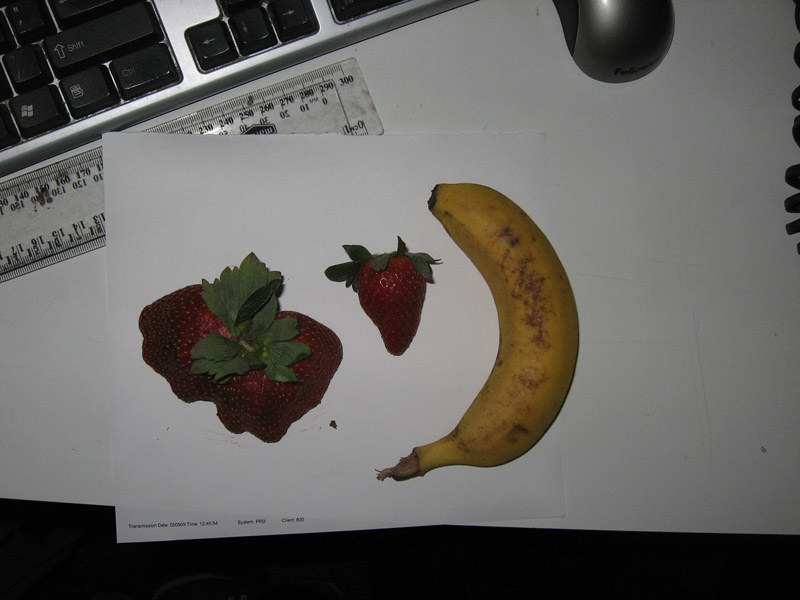On a white desk background, the top left corner of the frame features a silver computer keyboard with black keys. Just below the keyboard is a clear plastic ruler. To the upper right, a sliver of a silver computer mouse is visible. Slightly covering the clear ruler is a white piece of paper with a few letters at the bottom edge.

Centered towards the bottom of the frame, the right side of the paper hosts a semi-ripe, peeled banana. To the left of the banana, there's a strawberry hull with its stem still attached. Further left, a much larger deformed strawberry, resembling two fused strawberries, sits with its stem intact. The layout of these objects indicates a workspace setup with a hint of snacking amidst work.